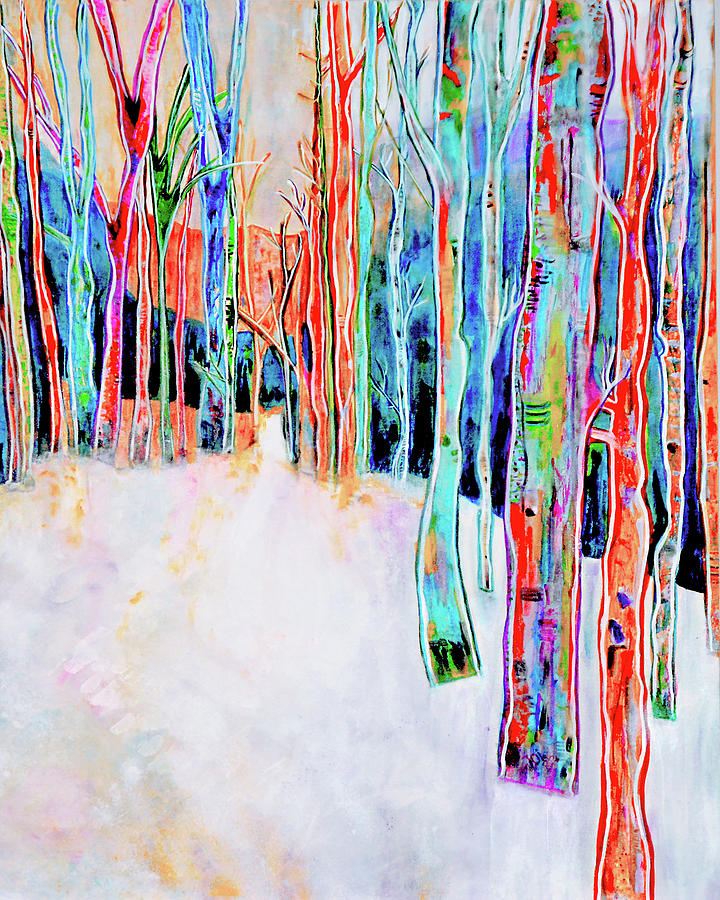The artwork is a vivid and abstract watercolor painting of a forest, featuring a lineup of neon and pastel-colored trees extending diagonally from the center to the right against a stark white ground. Each tree, distinguished by its bold outline of hues like turquoise, purple, pink, orange, red, yellow, and blue, stands out in this striking landscape. The branches and trunks are filled with various shades and complementary neon tones, lending an abstract and fluorescent quality to the scene. The minimal sky peeks through the dense canopy, while the ground is primarily white with subtle hints of purple and orange, creating a dynamic contrast with the vibrant trees. The dark background near the base adds depth to the composition, emphasizing the bright and whimsical nature of the trees. Overall, the painting exudes a striking balance and harmony through its use of colors and abstract form, creating a mesmerizing and visually engaging forest scene.